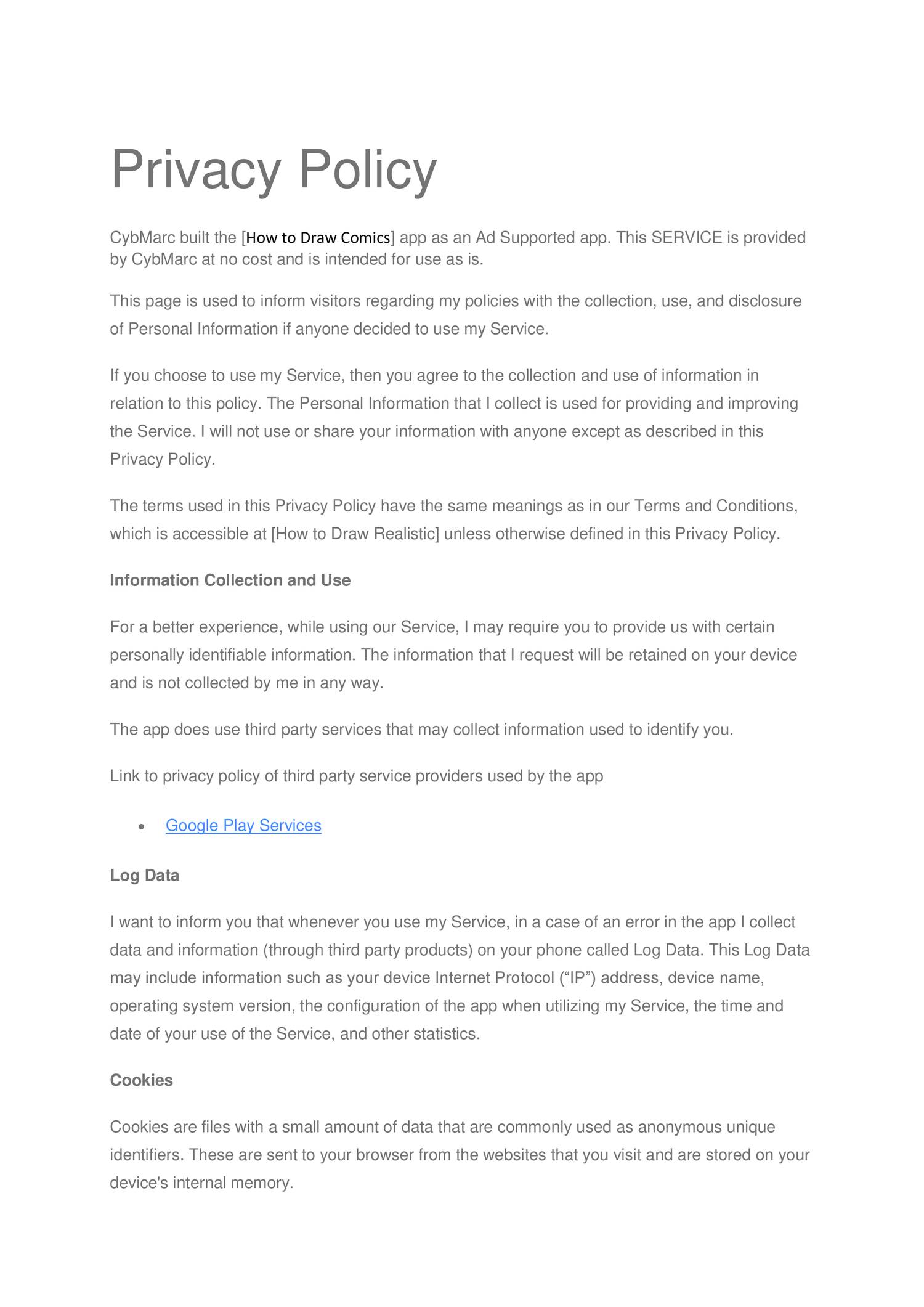*Civmark's "How to Draw Comics" App Privacy Policy*

This image displays the detailed privacy policy for the "How to Draw Comics" app built by Civmark. The app is offered at no cost and aims to provide a seamless user experience. The policy explains that the purpose of the page is to inform users about the collection and use of personal information when utilizing the Closer app.

Key points include:
- Personal information collected is solely for providing and improving the app’s service.
- Personal data is not shared or used beyond what is described in the privacy policy.
- The terms and conditions in this policy are consistent with those in other related documents.
- Essential information may be requested to enhance user experience, but no unnecessary data is collected.
- The app does not use third-party services to collect information; however, log data may be gathered through third-party products on the user's device.

Log data can include:
- Device and protocol address
- Device name
- Operating system version
- App configuration during use
- Time and date of service use

Additionally, the policy clarifies the usage of cookies and small data files, emphasizing they are not stored in the device's internal memory nor are they used to connect to the device.

This image serves to keep users informed about the privacy guidelines and data management practices employed by the app.